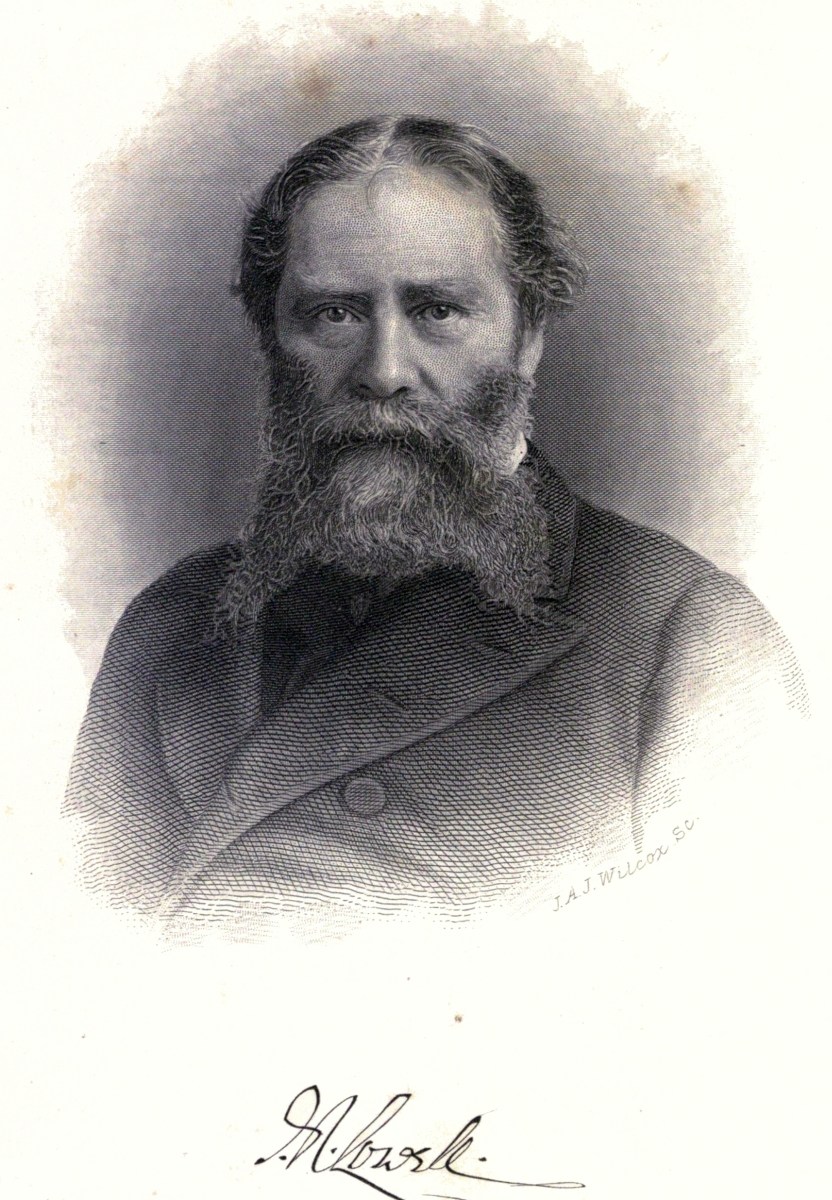This is a detailed and striking depiction of an older gentleman from the late 1800s or early 1900s, presented in a style reminiscent of wood prints or daguerreotypes. The image is in black and white, enhancing its historical feel. The man gazes directly at the viewer with a stoic expression, typical of the era when subjects had to remain still for long exposures. His wavy, curly hair is of medium length, and his facial hair is particularly notable: he sports thick sideburns, a handlebar mustache, and a very full beard that splits and extends downwards from the sides of his chin, leaving just stubble at the center. He wears a textured suit jacket that adds to the refined historical appearance. At the bottom right of the image, the name "J. A. J. Wilcox, S.C." is inscribed, likely identifying the artist, along with an unreadable signature beneath it.